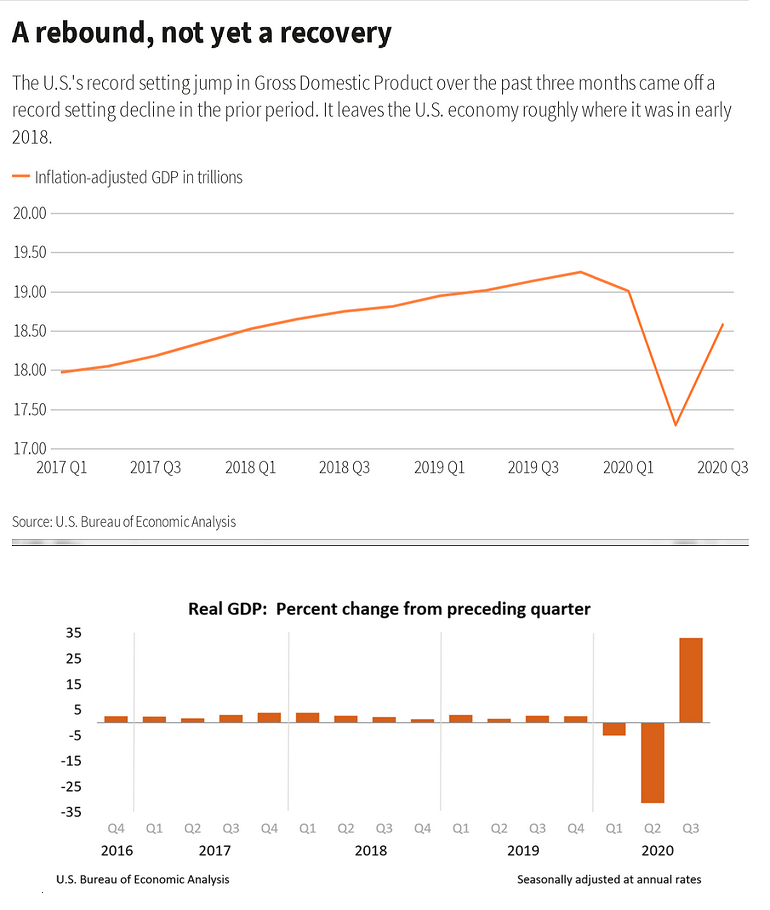The image features two graphs with the title "A Rebound, Not Yet a Recovery" at the top, which provides an overview of the U.S. economy's performance. The first graph, an orange line graph, is labeled "Inflation Adjusted GDP in Trillions" and spans from 17 to 20 on the y-axis and from 2017 Q1 to 2020 Q3 on the x-axis. This graph shows the U.S. GDP starting at a lower point in early 2017, rising steadily until peaking in 2019 Q3, then dropping sharply in early 2020 due to economic impacts before recovering partially by 2020 Q3, bringing the economy roughly back to its early 2018 levels. 

Below it, a bar graph titled "Real GDP Percent Change from Preceding Quarter" shows quarterly GDP changes from 2016 to 2020. The bar graph indicates minor, mostly positive growth until a dramatic decline in early 2020, followed by a significant rebound in Q3 2020. The y-axis ranges from negative 35% to positive 35%, illustrating the sharp contrast in economic performance across these periods.